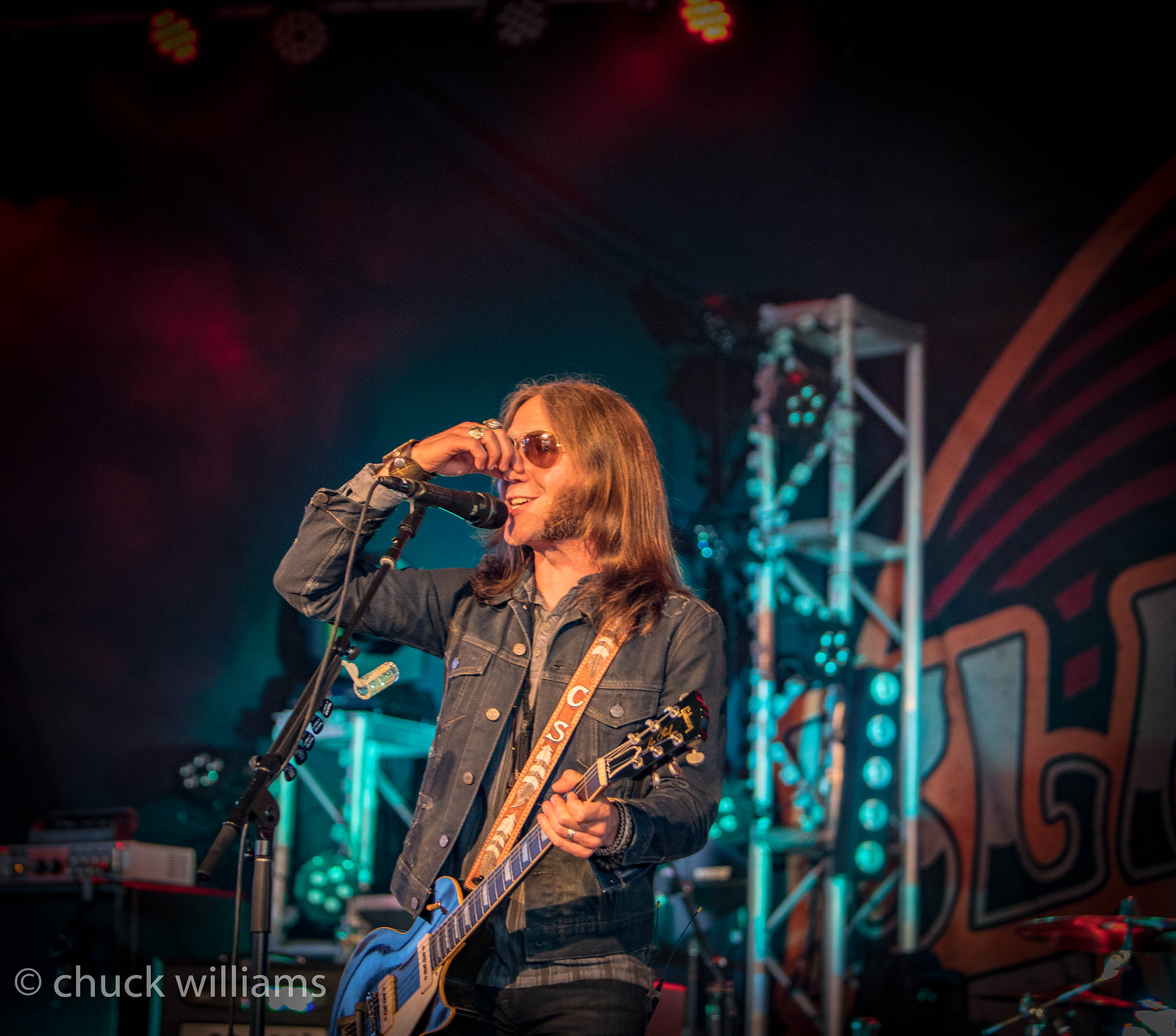The photograph captures a man standing on a stage, set against a dark yet colorful background featuring cloudy blues and reds with intertwined yellow and red decorations. Behind him, scaffolding adorned with silver, blue, and black lighting equipment is partially visible, as well as a symbol of a drum set. The man, positioned slightly off-center, holds an electric guitar and is dressed in a denim jacket, blue shirt, and dark jeans. His long brown hair flows around his face, which sports dark sunglasses through which his eyes are faintly visible, and distinct long mutton chop sideburns. He stands in front of a black microphone on a stand, his hand raised to his nose, adorned with two large rings. At the bottom left of the image, there's a copyright notice that reads "© Chuck Williams."